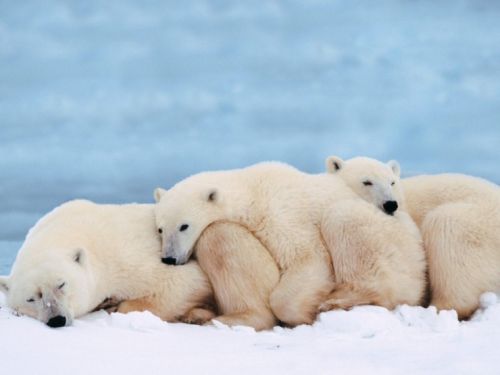In this captivating outdoor photograph, three polar bears are seen nestled together in a tranquil, snowy landscape, likely in the Arctic. Bathed in the soft light of day, the sky above displays a gentle blue hue with slight cloud cover, creating a serene backdrop. The polar bears, with fur that carries yellowish-tan and brownish tones in contrast to the pure white snow, exhibit black features on their inner ears, eyes, and noses, with a hint of gray around their noses.

Positioned almost in a horizontal line, the larger polar bear, presumed to be the mother, lies at the front with her head resting in the snow, as if dozing off. Behind her, one cub rests its head on her belly, and the second cub lies with its head on the first cub's back. The cozy arrangement, resembling a tender hug or a nap sequence, highlights a heartwarming scene of familial bonding amidst the wintry surroundings. The varying sizes of the bears reinforce the idea that the smaller ones may be the mother's well-grown cubs, each finding comfort in the warmth and presence of the others as they lie together in peaceful slumber.